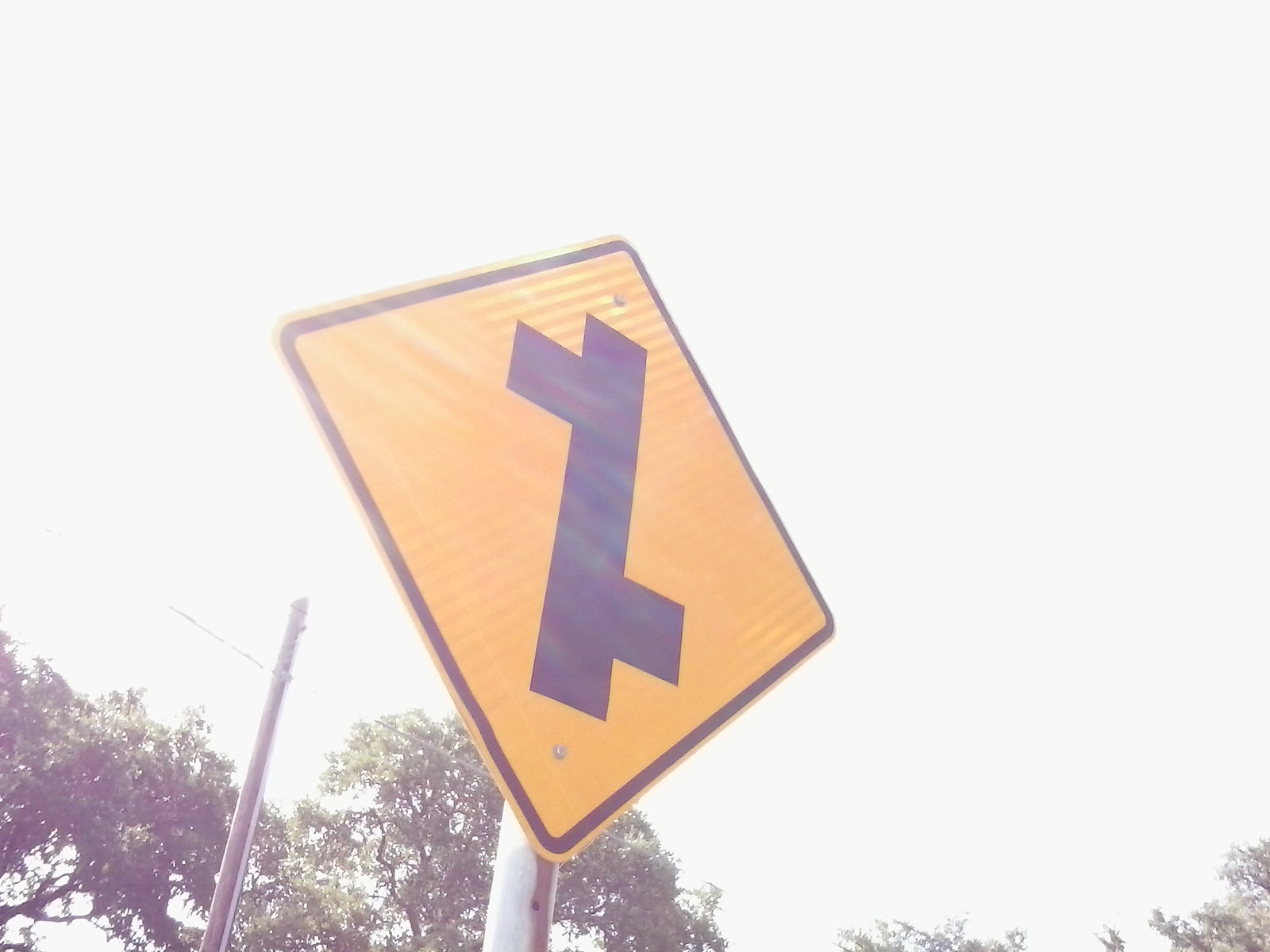In this photo, we are looking up at a road sign set against a very pale blue, almost white, sky. The road sign features a small gray pole at the bottom center, about an inch and a half high. On top of this pole sits a diamond-shaped sign with a black border and a darker yellow background. Inside the diamond, there is a detailed black symbol: a long, horizontal rectangle about four inches long and an inch and a half wide, with squares connected to its left upper side and bottom right area. The sign appears to illustrate intersecting roads, suggesting a road branching off to the right followed by another branching to the left. In the background, an electric pole with power cables stretches across, and the tops of some green trees are visible behind it.